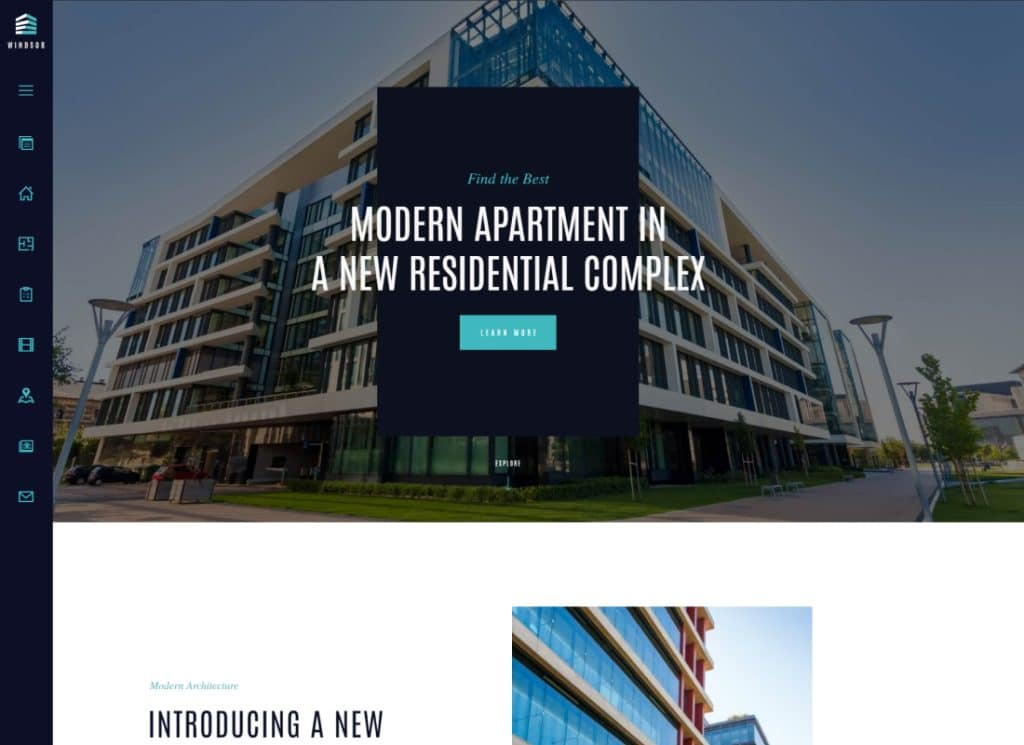This is an image of a website or possibly an app interface showcasing a modern apartment complex. On the left-hand side, there is a vertical navigation menu featuring various vector graphic icons. At the top left of this menu, there is a hard-to-read logo or symbol likely representing the website or app. Below the logo, the icons include three horizontal lines (likely a menu icon), a calendar, a home, a maze, a clipboard, a video clip, a map pin, a star on a rectangle, and an envelope.

To the right of this menu, there's a large hero image displaying an apartment complex with significant glasswork and numerous horizontal support lines. Centrally placed on this hero image is a black portrait rectangle containing white text that reads, "Find the best modern apartment in a new residential complex." There seems to be a teal button with white lettering below, although it is not fully legible.

Beneath the hero image, there is a section beginning with the phrase "Introducing a new," but the rest of the text is not visible due to the cut-off at the bottom of the screenshot. To the right of this section, there appears to be another smaller image showing a different view of the apartment complex.